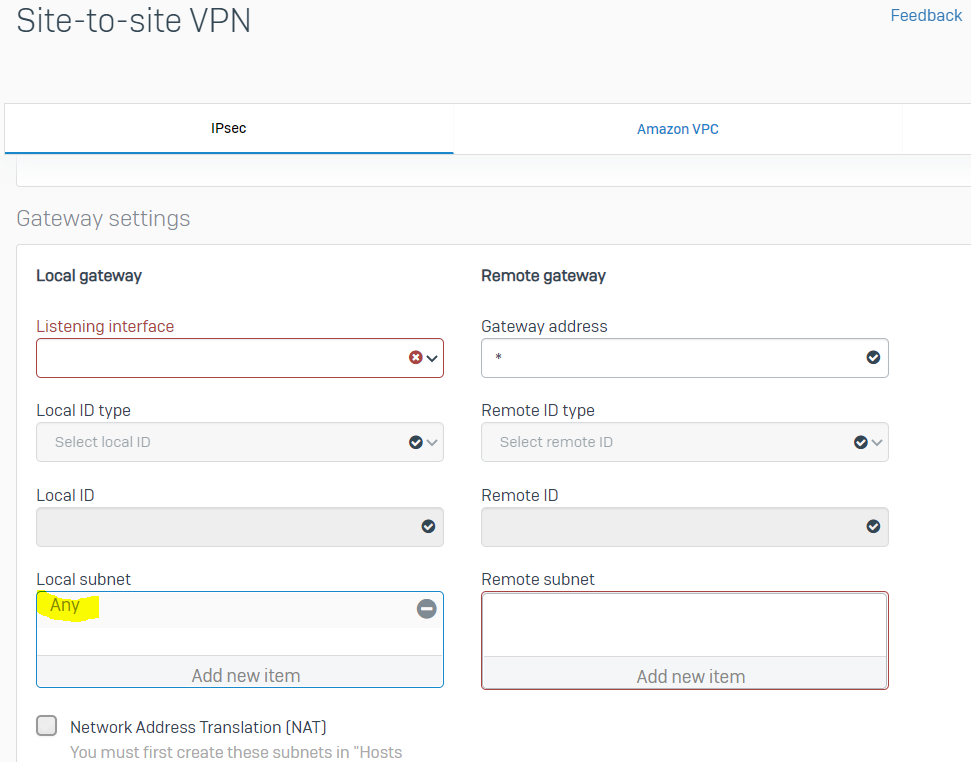The screenshot displays a detailed interface for setting up a Site-to-Site VPN. At the top of the interface is a banner labeled "Site to Site VPN." In the upper right-hand corner, there is a clickable "Feedback" link in blue, allowing users to provide their input.

Below the banner, the interface provides two clickable options: "IPsec" and "Amazon VPC."

A gray section titled "Gateway Settings" is displayed beneath these options, containing two columns for configuring VPN settings: "Local Gateway" on the left and "Remote Gateway" on the right.

Under the "Local Gateway" section, there are several fields:
- **Listening Interface**: This field is outlined in red, indicating it is a required selection, and users can click to choose their local listening interface.
- **Local ID Type**: A dropdown box where users can select the type of local ID. Currently, it has a checkmark but doesn't list the selected ID.
- **Local ID**: Also a dropdown box that is checked, yet no ID is currently displayed.
- **Local Subnet**: Highlighted in yellow, this field is currently empty, allowing users to add their local subnet information.

On the "Remote Gateway" side, similar fields are present:
- **Gateway Address**: For inputting the remote gateway address.
- **Remote ID Type**: Dropdown box for selecting the remote ID type.
- **Remote ID**: Input field for the remote ID.
- **Remote Subnet**: Field for adding the remote subnet.

At the bottom of the interface, a note about Network Address Translation (NAT) states: "You must first create these subnets and hosts before you do that." This indicates that subnet and host creation is a prerequisite for configuring NAT.

Overall, the interface provides a comprehensive and organized setup for establishing a Site-to-Site VPN connection.